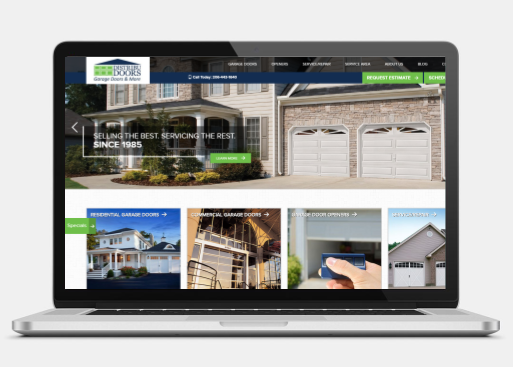This image is a low-resolution screenshot taken from a website called "Best Something Doors," viewed on a laptop or Chromebook. The primary focus is on a house featuring two elegant garage doors with slanted windows at the top, accompanied by the tagline, "Doing the best servicing the rest since 1965." The website interface displays several green clickable boxes, labeled "Learn More," "Specials," and "Request Estimate," among others. Additionally, smaller images on the webpage showcase various houses highlighting completed projects. The top section features a large house, while below, there are four smaller thumbnail images displaying more examples of the company's work.